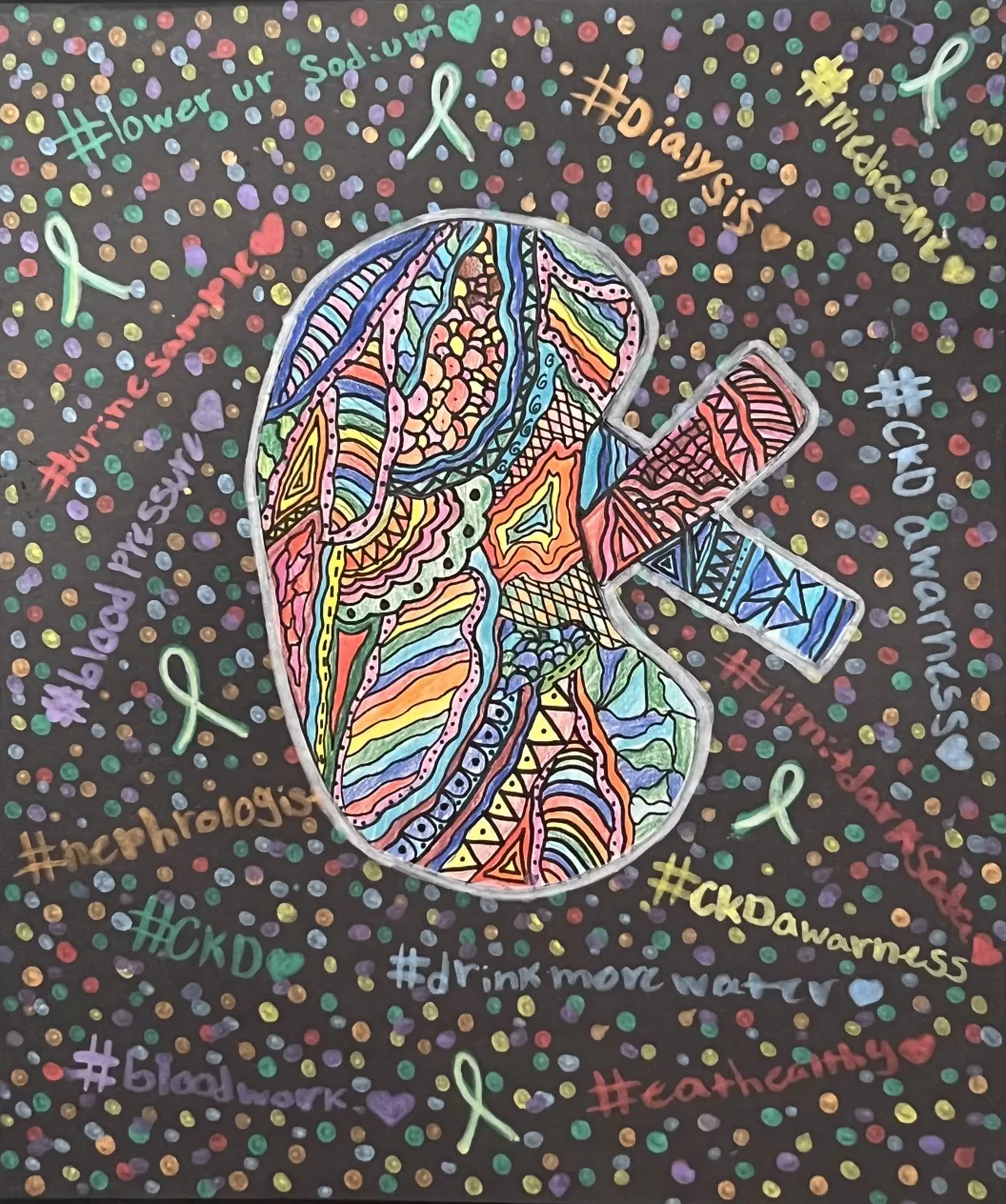The image is a vibrant, hand-drawn get well card focused on kidney health awareness. It features a black background peppered with multicolored dots and varied shapes. Dominating the center is a bean-shaped form resembling a kidney, adorned with intricate, paisley-like, optical art patterns in a kaleidoscope of colors, including greens, blues, reds, purples, yellows, and oranges. Emerging from the kidney shape are two tubular extensions: one extending to the upper right with intricate reddish patterns, and the other extending rightward with blue and black designs.

Surrounding this central kidney illustration are various hashtags written in different colors, adding context and highlighting key health messages. In the upper left corner, "#loweryoursodium" appears in green, followed by "#dialysis" with a heart in orange. On the upper right, "#medicare" also with a heart in yellow. The left side features "#urinesample" with a heart in red, "#bloodpressure" with a heart in purple, "#nephrologist" in dark green, "#CKD," and "#bloodwork" in dark purple. Below the kidney, there’s a light lavender hashtag, "#drinkmorewater." On the bottom and moving up the right side are "#eatyhealthy" in red, "#CKDawareness" in yellow, and another "#CKDawareness" in light lavender. Additionally, a barely legible hashtag amidst the dots reads "#limitdarksoda."

Overall, this card is a colorful, complex piece of art designed to convey messages related to kidney health through a mix of vibrant patterns and informative hashtags.